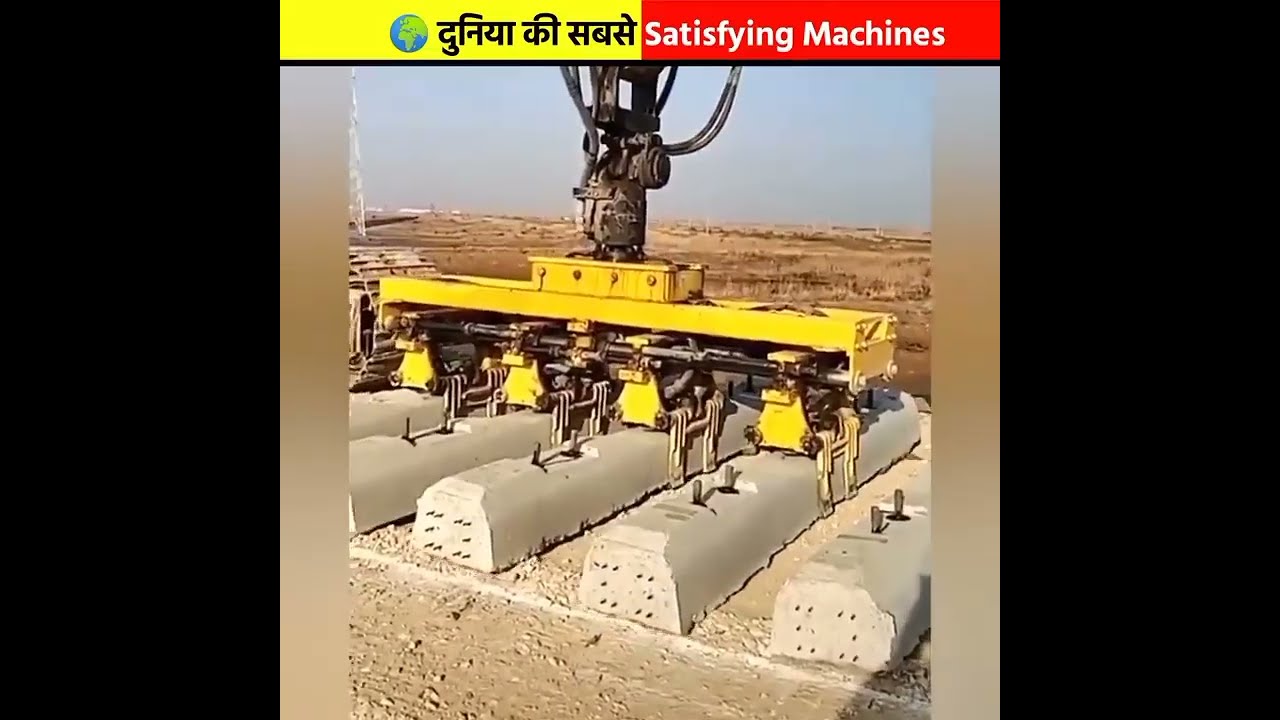The photograph captures a large, rectangular-shaped yellow machine positioned in a vast, dirt field reminiscent of a desert plain. This imposing machine features four distinct, octagonal compartments at its front, all supported by substantial, cement-colored stone logs. Above the main yellow section of the machine lies a black component festooned with wires, and from this section extends a steel or metal pole attached to various hydraulic systems. Further, a striking banner sits atop the image: its left side is yellow with black Arabic letters, while the right side is red with white text that reads "Satisfying Machines." This image appears to be a still from a video, with the top third showcasing a distant horizon and the entire scene bordered by black rectangles.